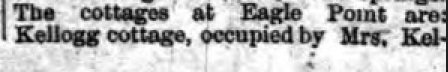The image is a small, rectangular clipping from what appears to be an old newspaper. The image measures roughly an inch in height by three to four inches in width. It features a grainy, off-white to grayish background. The text is black, resembling typewriter font, possibly Times New Roman, and cuts off abruptly on the right side. The clipping is bordered by a thin vertical pinstripe black line on the left side, which looks like it’s part of the newspaper print, and a definitive pinstripe black border on the right side. The printed text reads: "The cottages at Eagle Points are:" followed by a second line indicating "Kellogg Cottage, occupied by Mrs. K-E-L-", where the text is truncated. The overall appearance and the interruption of text suggest that only a portion of the original clipping is present.